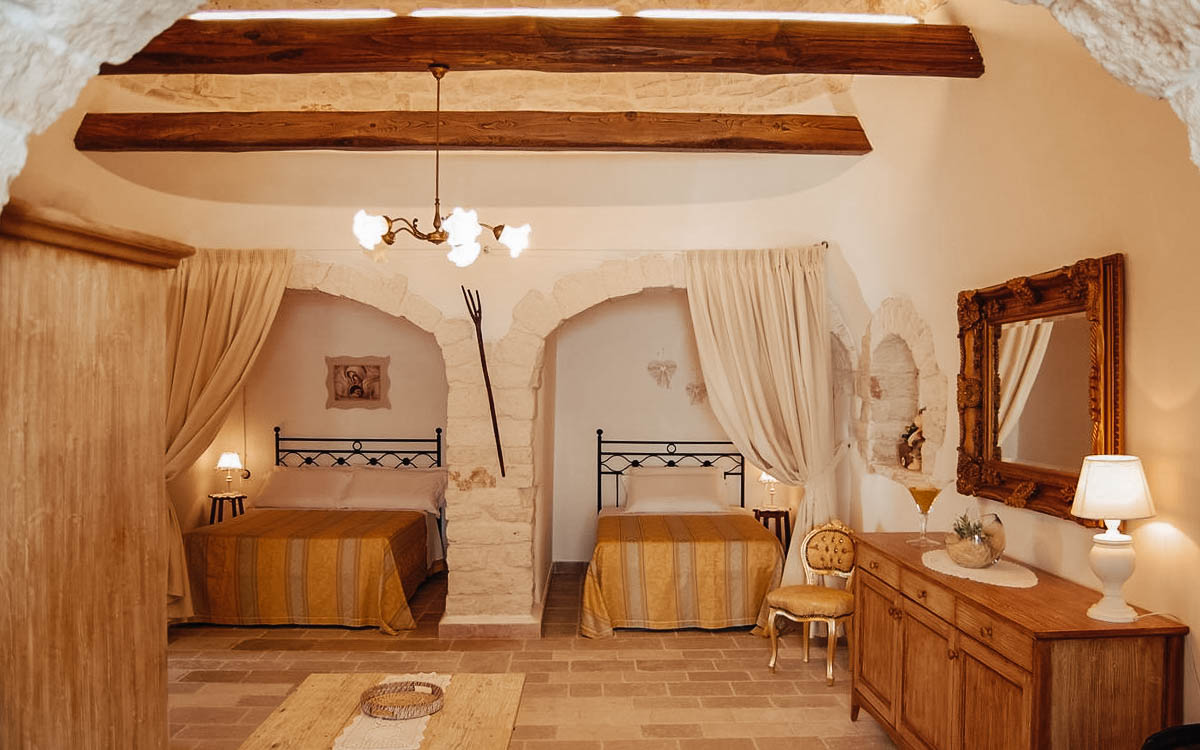This photograph captures a cozy, sepia-toned bedroom featuring a tan ceramic tile floor arranged in a brick pattern. The room is uniquely designed with two separate alcoves, each housing a bed beneath a rounded archway. The left alcove contains a double bed with a metal headboard, while the right alcove features a single bed with a similar headboard. Both beds have lights above them, illuminating the intimate spaces.

A central area of the room displays a dresser with a mirror, and a small desk on the right side of the room. The desk is adorned with a lamp and what appears to be a type of candle. An old-style chair reminiscent of the 1800s is situated below an additional archway on the left, which serves more as a decorative niche rather than a passage.

The ceiling showcases open wooden beams, adding to the rustic charm. There is also a curtain available to draw across the alcoves, providing privacy if needed. The room is well-furnished with not just beds but functional areas like the dresser and desk, creating a warm, inviting atmosphere.